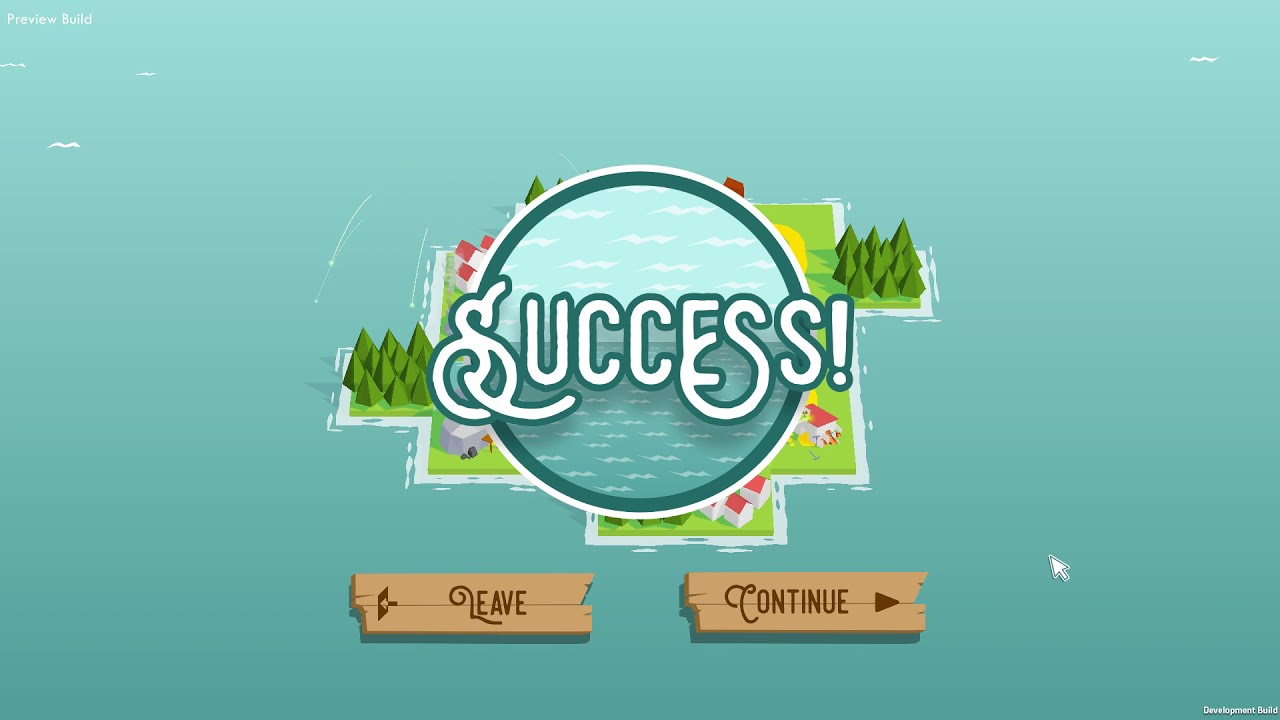In this detailed screenshot from a video game, the scene is set against a mostly light blue background. In the upper left corner of the image, there is text that reads "Preview Build." At the center of the image, dominating the composition, is a large aqua blue circle that features a cartoony depiction of an ocean with white-capped waves at the bottom and a sky with squiggly lines representing clouds at the top. Overlaid on this background is the word "Success" written in white cursive text. Within this circle lies a small, pixelated island composed of green squares, featuring several white buildings with red roofs and green, triangular trees.

Below the central circle, there are two wooden planks with text on them. The plank to the left reads "Leave" and the one on the right reads "Continue," each with respective directional arrows. The entire scene adopts a vibrant color palette that includes shades of white, light blue, dark blue, green, yellow, pink, red, brown, and tan, giving it a playful and engaging appearance typical of video game aesthetics. The design and elements suggest the user has successfully completed a level in what appears to be a puzzle game.